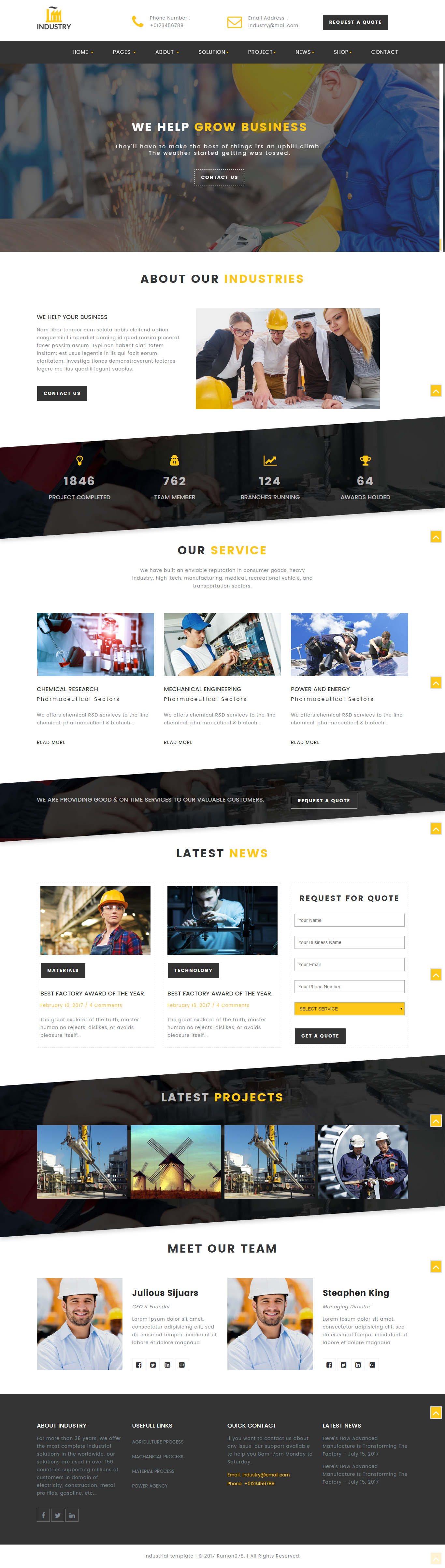Screenshot of a landing page showcasing business growth services, featuring the headline "We Help Grow Business" prominently. The page includes sections such as "Our Industries," "Our Services," and "Latest News." The screenshot captures a large, detailed view of the overall layout, though the icons and graphics are too small to read clearly. The design includes black and white bars arranged at angles across the page. The "Latest Products" section displays stock photos. There is global navigation at the bottom with a black background for the footer, adding to the overall professional aesthetic of the site.